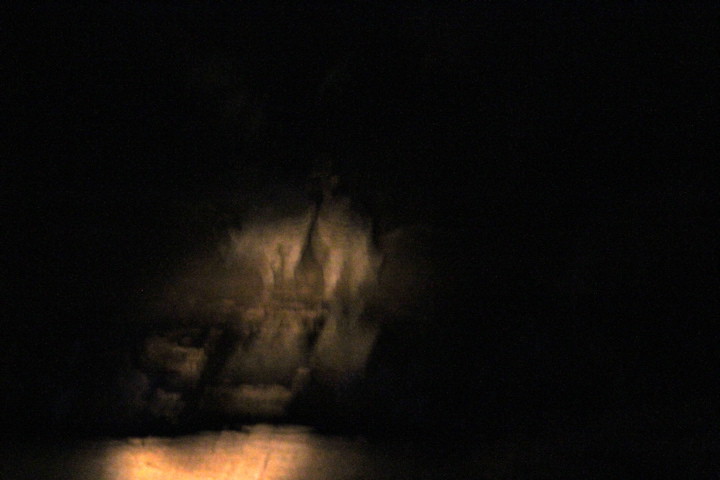The image depicts a very dark, highly blurry photograph that seems to be taken at night. The poor quality is marked by a significant amount of motion blur, fuzziness, and a grainy texture. In the otherwise pitch-black scene, a faintly illuminated area left of center reveals two extremely blurry figures, which appear to be either animals, possibly sheep or cows, or even wolves or dogs. These figures are described as being dark brown and white in color, with one seemingly looking to the right, and the other too blurry to determine. Green grass is partially visible around their feet. At the bottom of the image, beneath the figures, the light reflections hint at a possible pool of water, echoing the light source at the top.